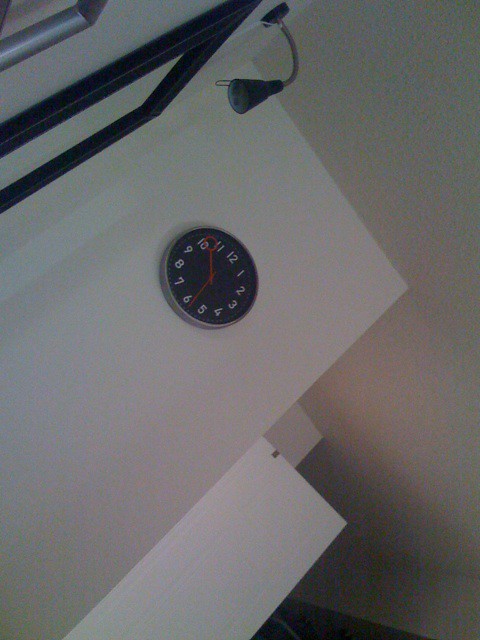The image features a black wall clock with a chrome outline, prominently displayed on a white wall inside a room. The clock face showcases Roman numerals for 6, 8, and 11, complemented by standard numerals for 1 through 12, ensuring the entire sequence from 1 to 12 is clearly visible. The clock has three hands: an hour hand, a minute hand, and a second hand. The simple yet elegant design of the clock contrasts subtly against the white wall, adding a touch of sophistication to the room's decor.